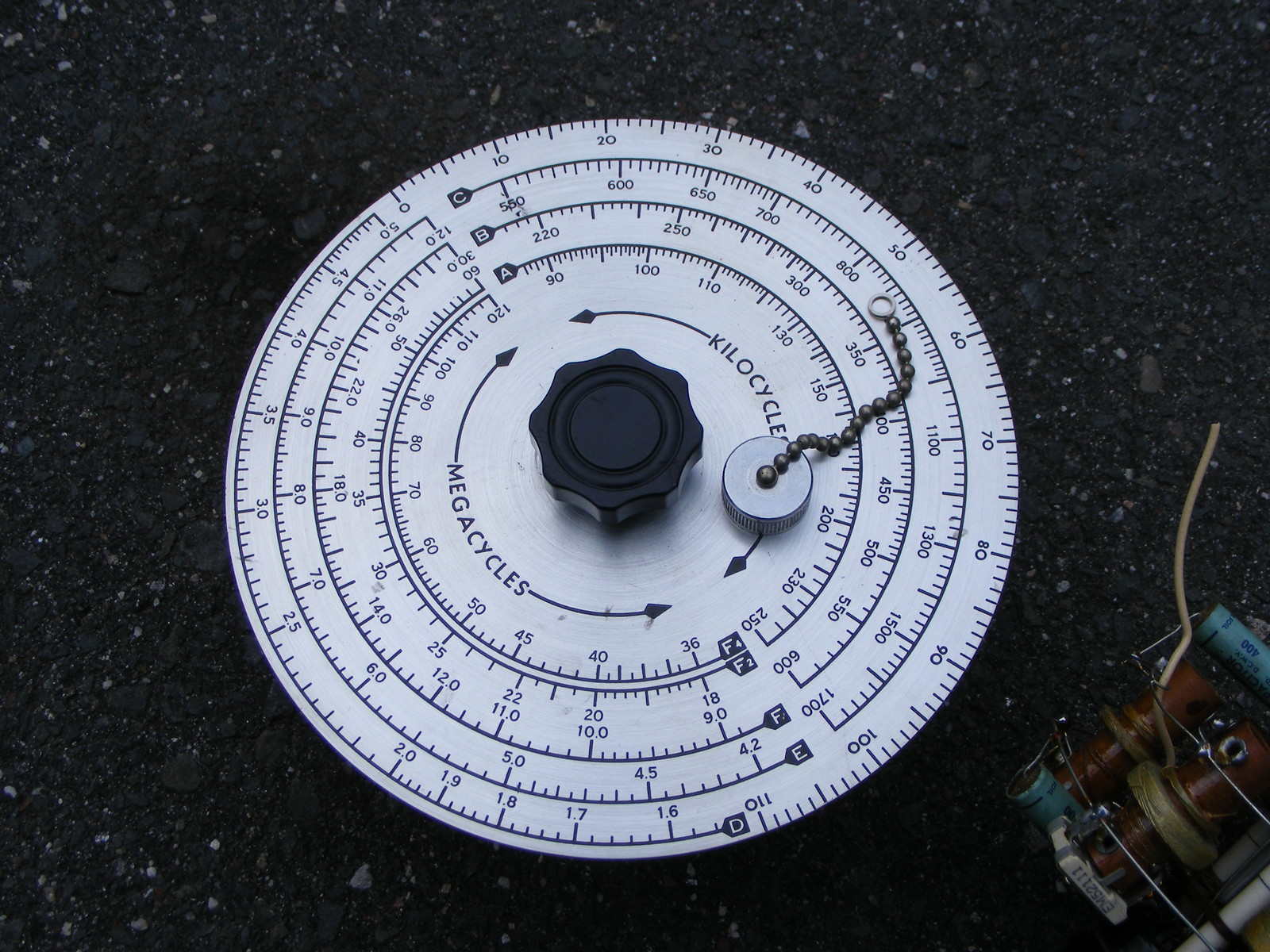The image captures a vintage radio frequency dial, characterized by a central circular interface with a whitish background. At the core of the dial is a small, black, rotatable knob used for tuning. Surrounding this central knob are six additional concentric circles, each marked with frequency measurements. 

The outermost ring is numbered from 10 to 110 kilocycles, increasing sequentially by tens. Another ring features megacycles with exact figures listed as 1.6, 1.7, 5.0, 11.0, 22, 25, and a range from 36 to 50. These concentric rings serve to assist the user in fine-tuning to specific frequency settings.

The dial rests upon a base of dark, rocky soil, adding a rustic touch to the image. To the right of the dial, there is an object that resembles an old battery pack, colored in a worn brown hue with patches of blue on its sides, where one can see batteries protruding.